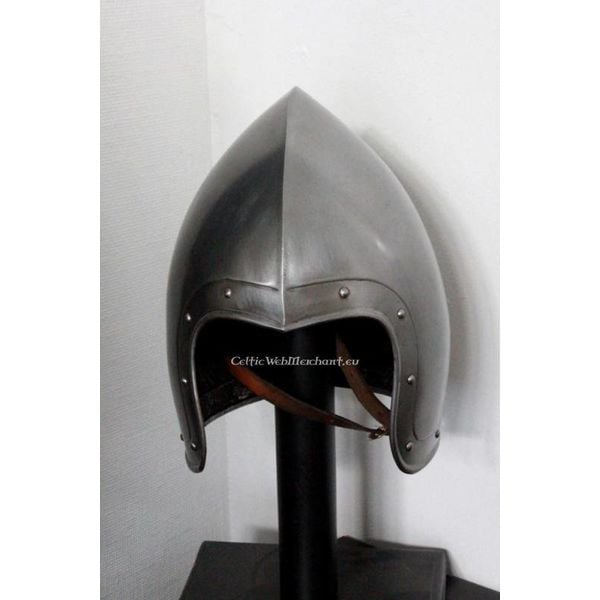The photograph features a medieval or Renaissance era helmet, crafted from silver-gray metal with a pointed, spear-like top. The helmet has a series of bevels and eight small studs around the face opening, which add to its ornate design. Inside the helmet, a brown leather strap is visible, likely used for securing it on the wearer's head. The helmet is displayed on a black stand with a two-inch diameter tubular support, mounted on a black square base that sits on a small table. The background is white, suggesting it is placed in the corner of a room. At the top of the image, the URL "CelticWebMerchant.eu" is displayed in white, italicized text, indicating the source of the photograph.